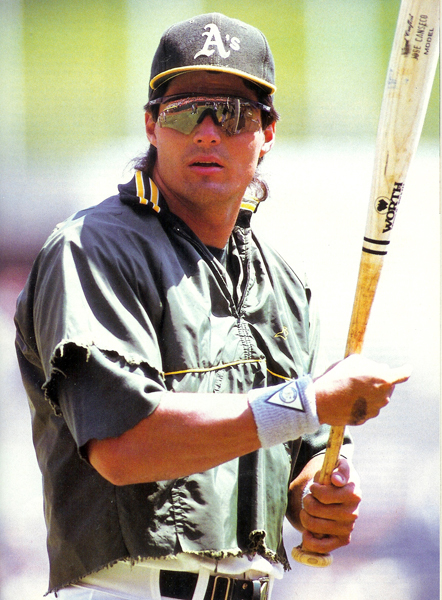The photograph features a baseball player, possibly a young Jose Canseco, decked in a characteristic ensemble. He wears a black baseball cap with a yellow brim, emblazoned with a large white "A's" on the front. His eyes are shielded by black-rimmed, silver-lensed reflective sunglasses, and his long hair, styled in a mullet, flows beneath the cap. He is dressed in a sleeveless black vest with frayed edges on both the sleeves and bottom hem, layered over a white baseball jersey. His lower attire includes white pants secured with a black belt featuring a silver buckle. He sports a fabric wristband with a white triangle on it. In his left hand, he grips a wooden bat labeled "Worth," which shows signs of a white substance applied midway up the bat. The setting is indeterminate due to the heavily blurred background, though a hint of a flag suggests it to be a typical baseball environment. Despite the potential bruise visible on his right hand, he faces the camera with a steady gaze.